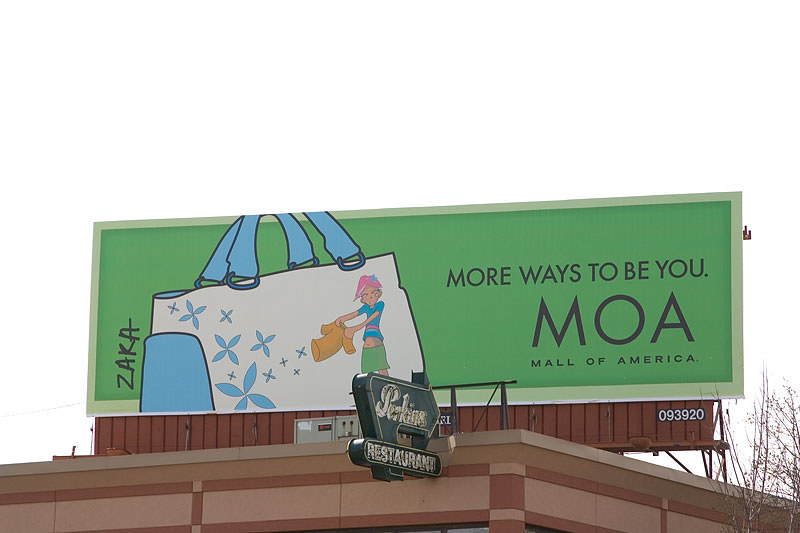This image features a large rectangular billboard perched atop the flat roof of a building. The building itself is painted in a combination of pink and sandy hues. The rooftop prominently displays a sign that reads "Perkins Restaurant," suggesting it is an establishment within or adjacent to the building.

Dominating the scene, the billboard is vibrant green and showcases a shopping bag. On this bag, there is an illustration of a woman shaking out a shirt, with several 'X' symbols emanating from it. The billboard carries the slogan "More Ways To Be You" in bold text, accompanied by "MOA" and "Mall of America" in very large letters, clearly identifying the advertiser. This vivid advertisement likely serves to promote the Mall of America, indicating the diverse shopping options and experiences available at the mall. The juxtaposition of the Perkins Restaurant sign and the Mall of America advertisement suggests that the location is either part of the mall or situated within close proximity to it.